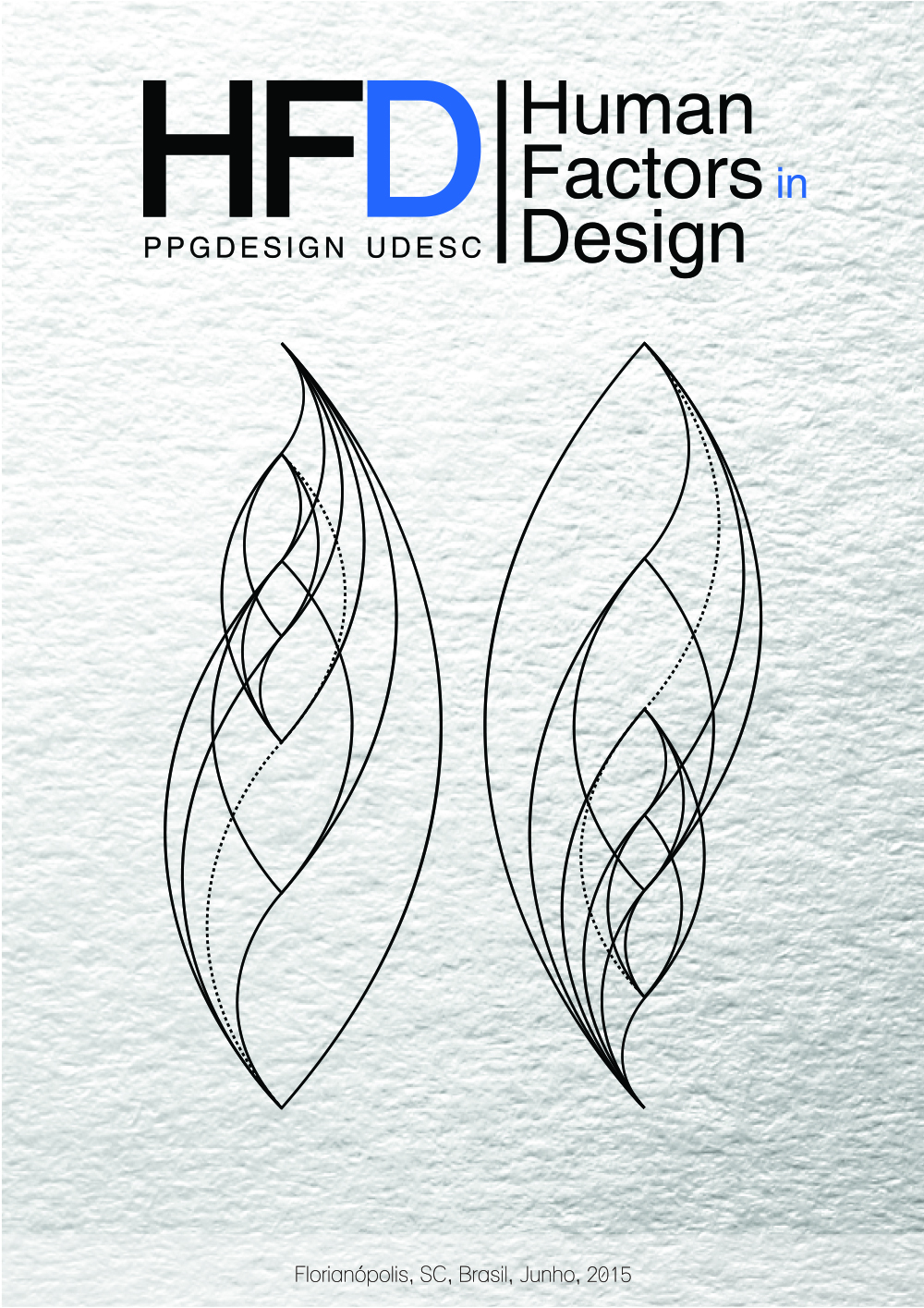The image is a vertical rectangle, possibly a book cover or a poster, related to human factors in design. It features a textured white background with a grayish tone. Dominating the top center are the large letters "HFD," with "H" and "F" in black, and "D" in blue. Below this, the text "PPG design UDESC" is prominently displayed, with a dividing line beneath it leading to the phrase "human factors in design," where the "N" in "human" is notably blue, contrasting with the otherwise black text. Central to the design are two vertical, leaf-shaped objects composed of smooth, curved lines and dotted lines, arranged as reciprocals of each other, one ascending from the bottom and the other descending from the top. At the very bottom, in very small print, the text reads "Florianopolis SC Brazil Junho 2015." The overall layout and visual elements suggest a clean, modern design focus without the inclusion of photographs, emphasizing the subject of design principles.